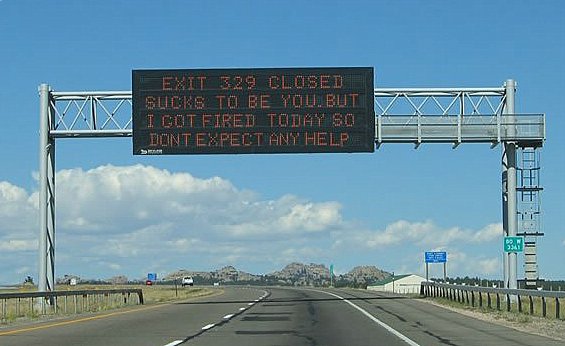On a clear day with blue skies and a few scattered clouds, a two-lane interstate highway stretches into the distance. A steel frame structure spans across the lanes, supporting a large black electronic sign that reads in bold, red letters: "Exit 329 closed. Sucks to be you, but I got fired today, so don't expect any help." The structure is positioned above the road where white dotted lines divide the lanes, with continuous white and yellow lines marking the sides. To the right of the highway, a blue sign and a green sign are visible near a guardrail. Behind these signs, a building with a green roof and white exterior can be seen. In the horizon, majestic mountains rise, enhancing the scenic vista. The highway median is adorned with a strip of grass, adding a touch of greenery to the landscape, as the road gently curves away from the sign.